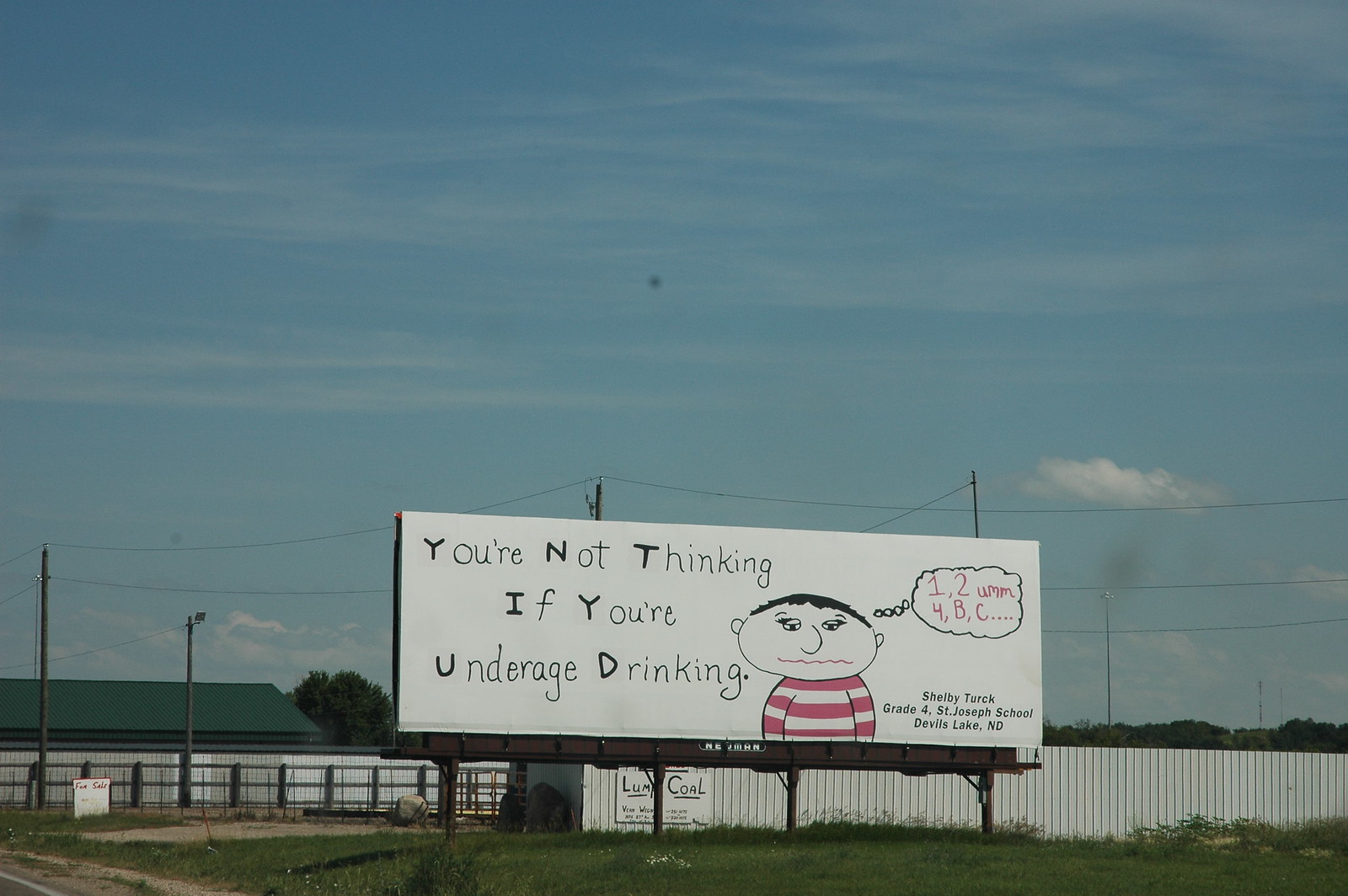This outdoor photograph captures a relatively low, white billboard elevated a few feet off the ground on a dark brown or black frame with four legs. The billboard, designed to discourage underage drinking, prominently displays the black, bold-lettered message: "You're not thinking if you're underage drinking." To the right of this text is a simple cartoon of a child, likely a boy with dark hair, wearing a red and white striped shirt. The boy appears to be thinking, evidenced by a thought cloud that says, "one, two, um, four, B, C, dot, dot, dot.” At the bottom right of the billboard, there's an attribution: "Shelby Turck, grade 4, St. Joseph School, Devils Lake, North Dakota," suggesting this is part of a school project. Surrounding the billboard are details that place it at the edge of a field: a white fence, an additional fence with brown or dark gray posts, power lines, a blue sky with a few clouds, a row of trees on the horizon, and a house with a green roof to the left.